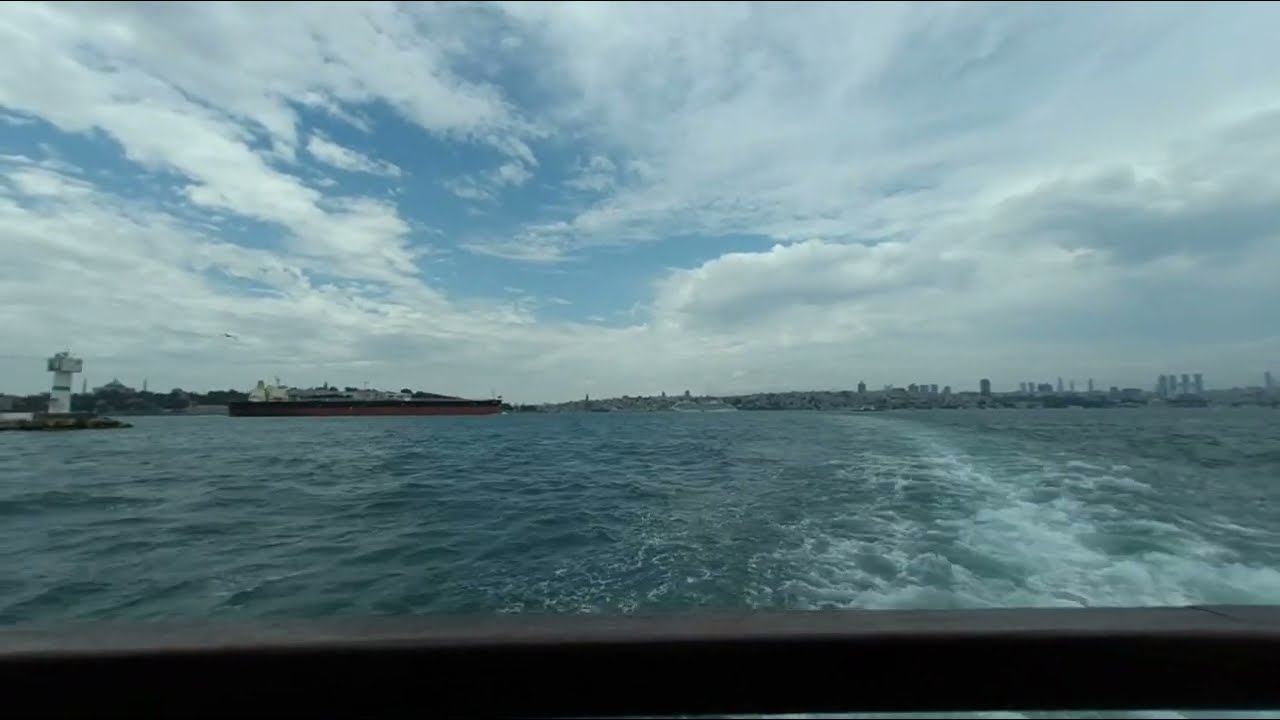This photograph captures the view from the back of a sizeable boat, suggested by the prominent wake frothing behind it. The scene depicts a large bay or waterway with choppy, dark blue water, stirred into waves by the boat's motion. A brown wooden railing is visible at the bottom edge of the image, confirming the perspective from the boat. The sky above is overcast and gray, filled with numerous clouds, although patches of bright blue sky break through in places. To the left, there is a long, red and black barge docked near the shoreline, and some trees and buildings are dotting this side. The right side of the horizon reveals the distant edge of land, speckled with high-rise buildings. The overall impression is of a hazy, potentially stormy day over an urban waterfront.